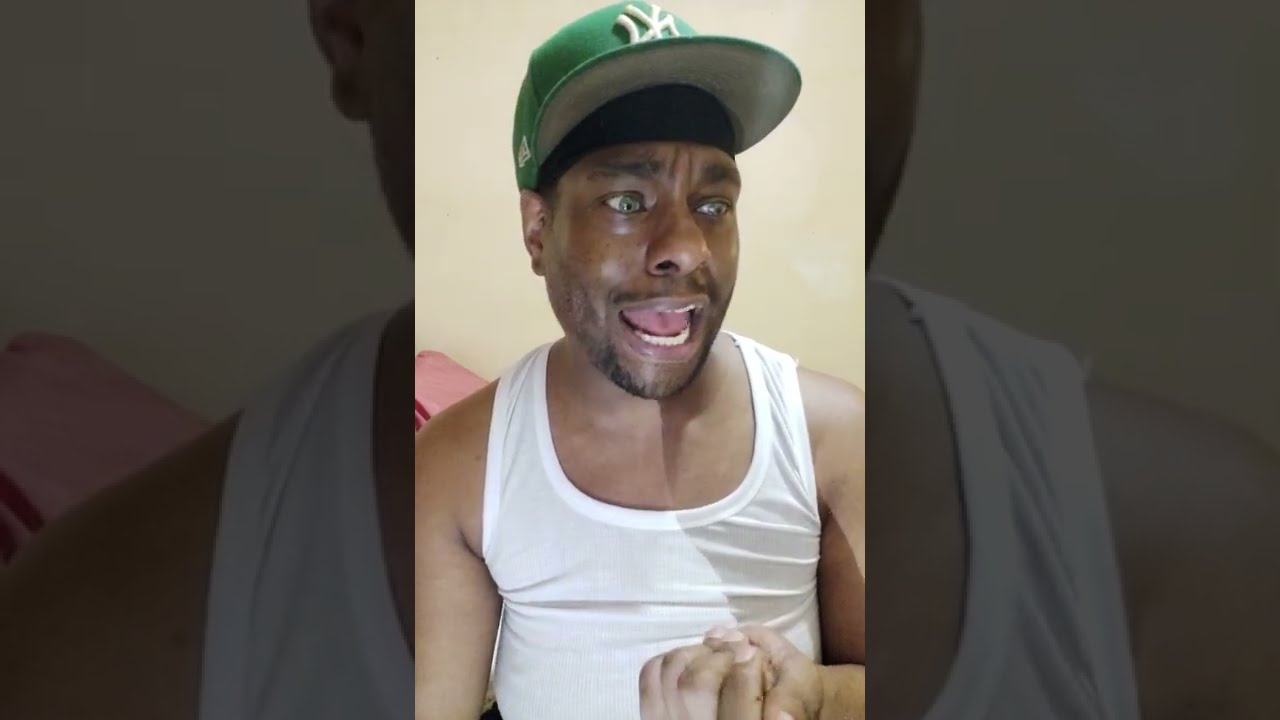The image consists of three frames centered around a main photograph of an African American man, Kent, who is wearing a green and white New York Yankees baseball cap with an obscured logo and a sleeveless white tank top. The central frame captures Kent making an expressive face, possibly in surprise or discomfort, although it appears he might just be playing around. His mouth is open as if he is speaking, and he has a slight amount of facial hair. His head is turned slightly to the left, and his left arm is extended with his fist in front of his torso. On the lower right of the image, his hand is visible. The left and right panels are dimmed or underexposed enlargements of sections of the central image, adding an artistic, fragmented framing effect to the photo. The composition suggests an engaging and dynamic moment caught on camera, possibly during a casual recording session.